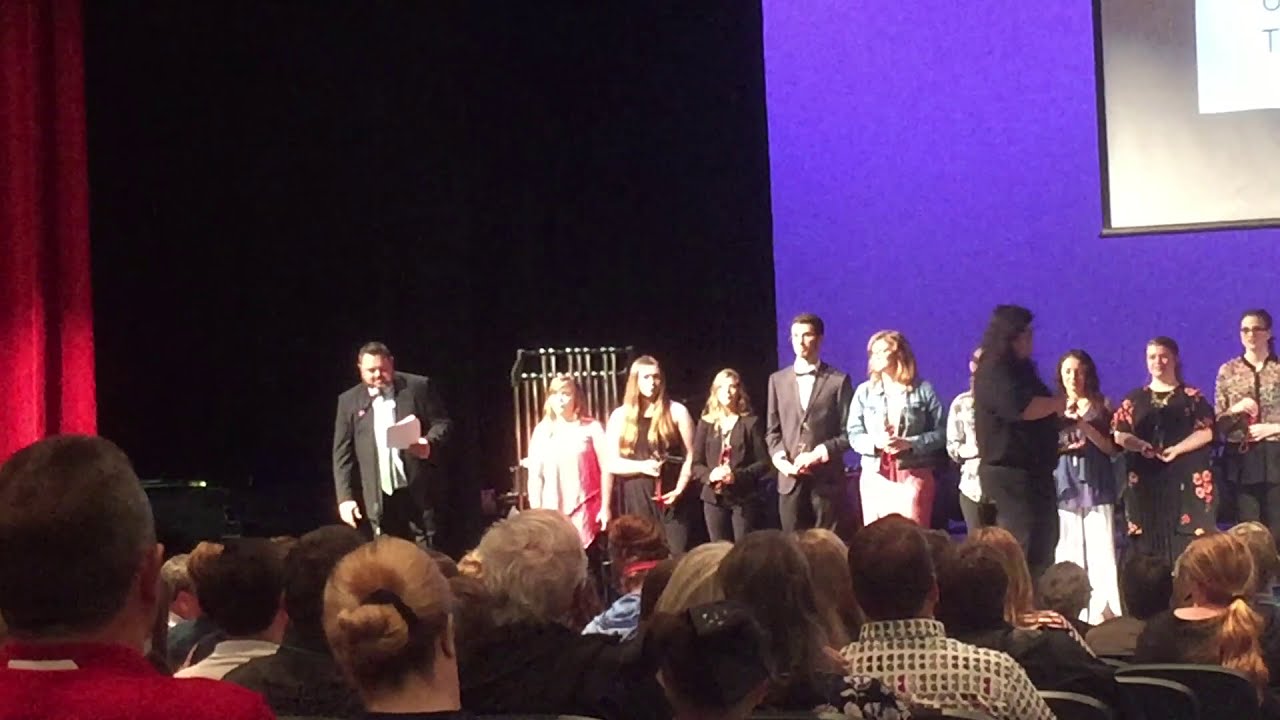The image depicts a high school award ceremony or celebration in a large auditorium. On the stage, a man in a black suit with short hair is reading from a piece of paper into a microphone on a stand. In front of him, 8 to 10 high school-aged individuals stand shoulder to shoulder, dressed in semi-formal attire. Some are holding trophies or ribbons. Notably, the stage has a backdrop that is part black and blue, with red curtains. There's a projector screen in the background displaying a white slide with black and gray borders and partial text visible. The audience, seen only from the back of their heads, fills the foreground, seated and facing the stage. The atmosphere suggests a formal school event with students being recognized for their achievements.